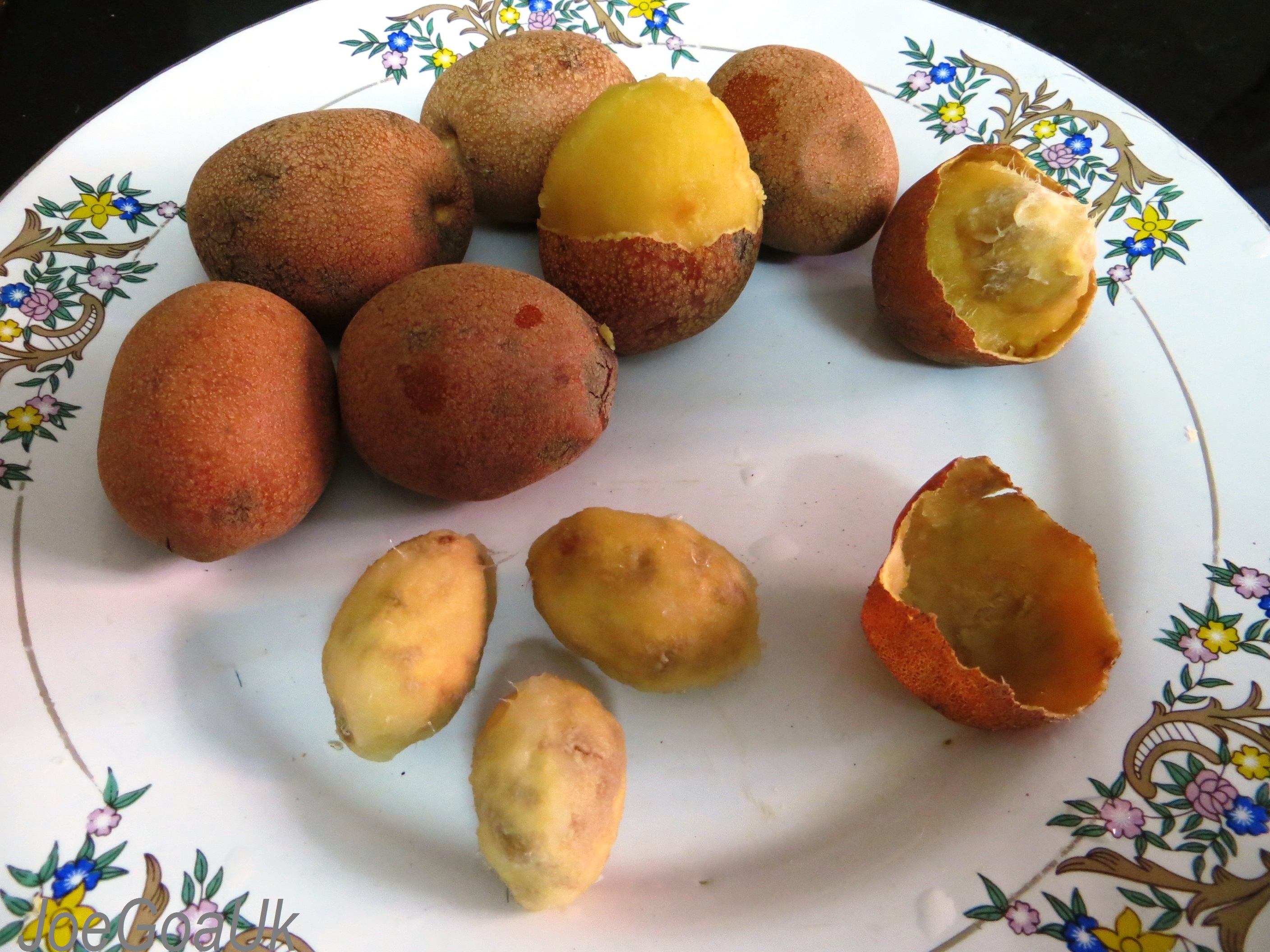This horizontal-rectangular photograph showcases a pristine, white circular plate adorned with a detailed floral design featuring alternating patterns of gold rings, pink roses, blue flowers, yellow daffodils, and green leaves, all connected by a delicate line. The plate holds ten cooked potatoes, some with a red skin and others with a light brown skin. Among them, three smaller potatoes are fully peeled, two are partially peeled, and five remain intact. Visible pieces of potato skin are scattered on the plate, accentuating the preparation process. The background is a stark black, which adds a contrasting depth to the vibrant details of the plate and potatoes.